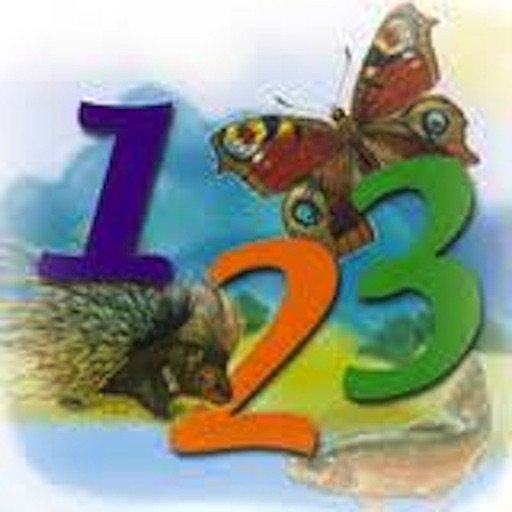This blurred image appears to be a colorful illustration, potentially from a children's book, featuring the numbers 1, 2, and 3 arranged in a staggered fashion. The number 1, depicted in ocean blue, rests higher than the others and is positioned on the back of a dark-colored porcupine, which appears to be sniffing the orange number 2. The orange number 2 is the lowest in position and is being bitten by a small fox or animal of some kind. The green number 3 stands partially higher than the 2 but lower than the 1, adorned with a butterfly with red and gold wings resting atop it. Set against a backdrop of blue mountains and a light blue body of water, there's a fish visible in the water, darker on the top and lighter on the sides, resembling a light brown or salmon color. This vibrant, yet slightly unfocused scene, contains no date or specific identifying information, giving it a timeless, whimsical quality typical of storybook illustrations.